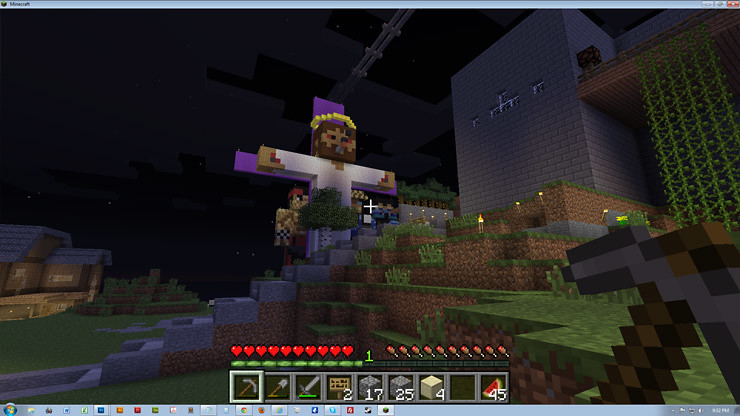This detailed screenshot captures a moment from a video game played on a Microsoft desktop computer. The distinctive Microsoft logo is prominently visible, along with the recognizable bottom taskbar filled with open applications such as Google Chrome and Steam, among other system icons. The upper section of the screen features a banner with standard window control symbols including the close (X), minimize, and expand icons. In the top-left corner, the Microsoft name is clearly displayed.

The central focus of the image is a scene from a Lego-themed video game, characterized by its unmistakable blocky, pixelated aesthetics which mimic the iconic Lego style. Dominating the scene is a Lego representation of Jesus on a purple cross, situated in the middle of the image. Lego Jesus is depicted wearing a white garment and a gold crown. 

In the foreground, there is a green, grassy hill with stairs leading up to the crucifixion scene, providing a pathway to the central figure. The background showcases a gray brick building, emphasizing the constructed, model-like environment typical of Lego worlds. Overall, the screenshot offers a unique blend of religious iconography and playful, Lego-based digital recreation.